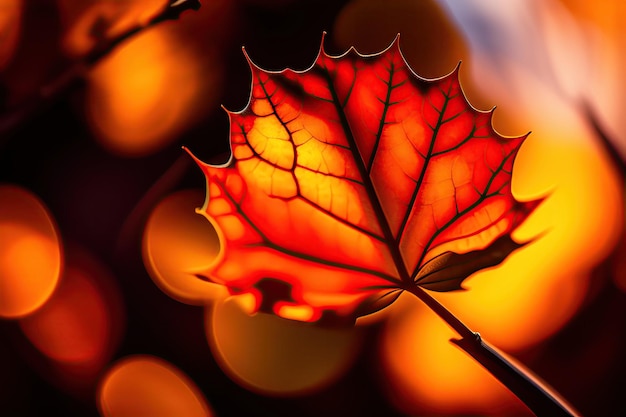This image depicts a close-up, CG-rendered leaf that is predominantly orange with streaks of amber yellow and brown. Its shape is round with sharply spiked, jagged edges and elongated points extending outward. The central brown stem branches into a network of black veins that radiate throughout the leaf. The background is heavily blurred, featuring a bokeh effect with black as the primary color, accented by glowing orbs of orange arranged in a diagonal pattern across the lower left and parallel to another series of three orbs. The entire scene has a smoky, ethereal glow, giving the impression of an illuminated leaf against a dark, yet vibrant, backdrop.